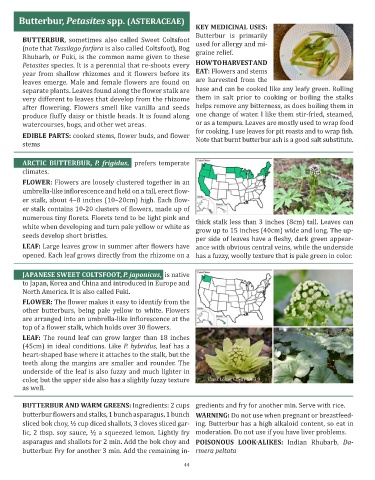This image appears to be a detailed page from a plant identification guide or textbook, showcasing various edible plants and their optimal growing regions in the United States. The page is divided into three sections, each focusing on a different plant: Butterbur petasites SPP, Arctic Butterbur, and Japanese Sweet Colt's Foot. The sections are titled in dark green text, with the headers distinctly separating the content. 

Each section includes descriptions of the plants' flowers, leaves, and sizes, along with specific details about their edible parts and medicinal uses. The Butterbur, for instance, highlights that its stems, flower buds, and flower stems are edible. The accompanying text provides guidance on how to eat and harvest these plants. 

To the right of the descriptions are photographs of the plants for visual identification, also bordered in green, along with a map of the United States marking the regions where these plants can be grown, primarily in the northwest and northeast. The overall color scheme of the page combines white text and imagery with green accents and black outlines, making it visually cohesive yet somewhat challenging to read due to the color contrast.